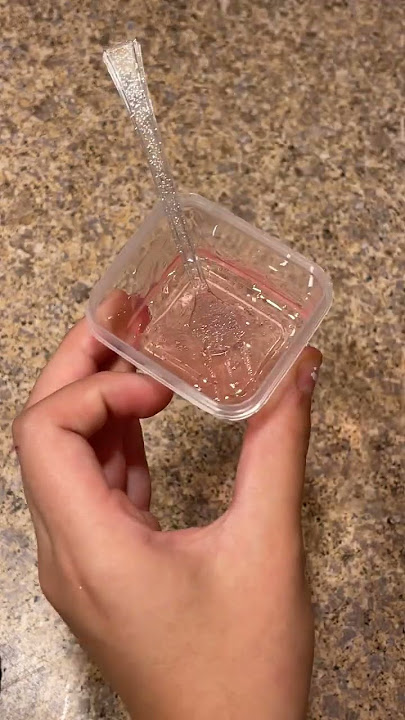This color photograph, taller than it is wide, features a left hand of indeterminate gender and fair skin holding a small, square, clear plastic container over a brown, gray, and black speckled granite countertop. The container holds a pale pink, clear gelatinous substance. A shiny plastic fork is embedded in the gelatin, angled upwards with its handle toward the top left corner of the picture. The fork has white sprinkles on it and features two distinctive lines running down the sides of its prongs. The hand grips the container with the thumb and three fingers, while the index finger is bent slightly for support. Outside of the hand and container, no other people, animals, or structures are visible in the image.